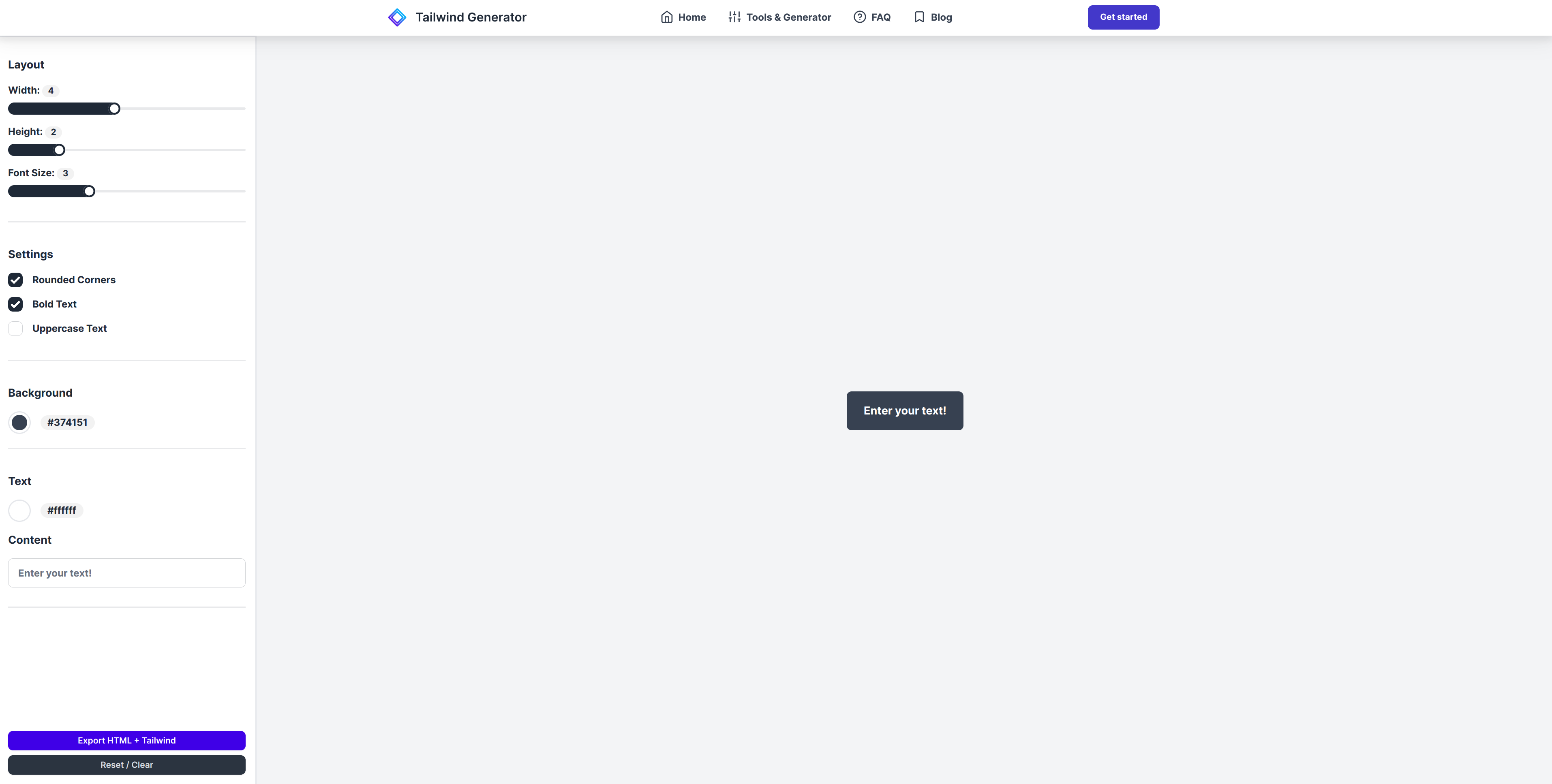The image is a horizontally rectangular screenshot displaying the interface of a web-based tool. The screen is divided into sections with a white background on the left-hand side and top, and a light gray background occupying the remainder. The left white section, in a vertical rectangular shape, houses various options for customization, including layout settings with three sliders labeled for width, height, and font size. Below the sliders are settings options, two of which are checked: "Rounded Corners" and "Bold Text." The third option, "Uppercase Text," is not checked.

Further down, there are sections labeled "Background," "Text," and "Content." Under "Content," there's a text field where users can input their information. At the bottom of this section are two small buttons; however, the text within them is too small to be legible in the screenshot.

The white area at the top displays the navigation and header options: "Tailwind Generator," "Home," "Tools and Generator," "FAQ," "Blog," and a prominent purple "Get Started" button.

The larger portion of the image with the light gray background features a single button centered in the frame, which reads "Enter Your Text."